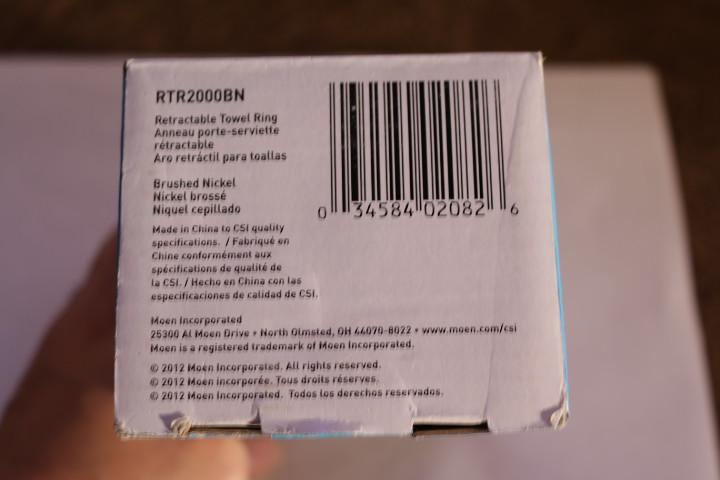This image features a close-up, zoomed-in view of a box package. In the upper left corner of the package, there is a stock number. Directly beneath the stock number, text indicates that the product inside is a "retractable towel ring," with the same information provided in multiple languages. Centered slightly to the left and below the initial text, the package details the product specifications, noting that it has a brushed nickel finish. Again, these details are translated into various languages. Additionally, there is text stating "Made in China" and some other specification-related information.

This product is manufactured by Moen, a detail accompanied by the company's name and address. Trademark information is located in the upper right corner of the package. A barcode is also present. The perspective of the image suggests the viewer is looking down at the top of the package. Surrounding the package is a white surface area and a darker wall in the background.